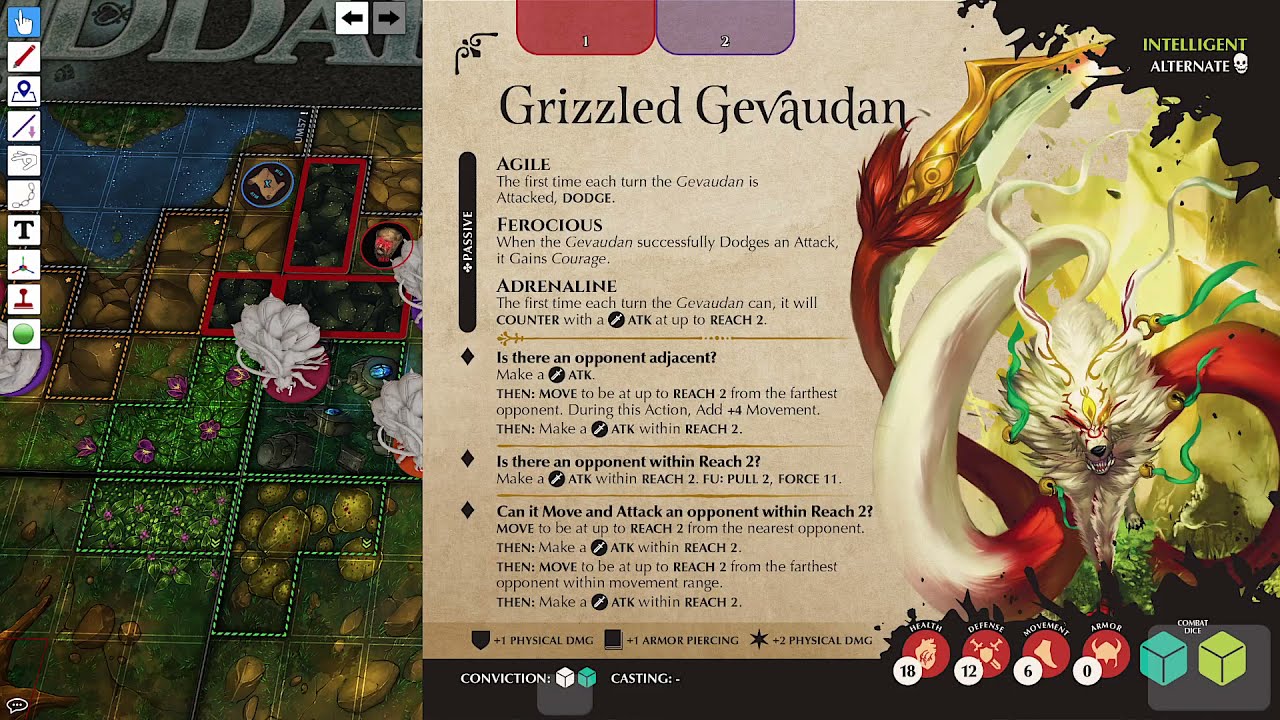The illustration depicts a video game, likely a strategy or role-playing game, with a highly detailed interface. On the left side, there's a vertical column featuring a variety of icons, starting with a finger pointing upward, followed by a pencil, suggesting some drawing or custom input functionality within the game. This section of the game interface may serve as a palette or menu for drawing tools, enhanced by the presence of various buttons resembling those in an art application.

Dominating the central area of the illustration is a piece of paper or document with the title "Grizzled Gevaudan," providing instructions or character attributes such as "Agile," "Ferocious," and "Adrenaline." It includes specific gameplay instructions like assessing whether an opponent is adjacent or within a certain range. This document is accompanied by a grid-like background with multiple decorative elements, including flowers and what appear to be food-related items like eggs.

On the right-hand side, there's a notable image of a creature resembling a lion or wolf, featuring a large tail adorned with a metallic element at its end. This creature appears to be in motion, enhanced by wave-like graphical effects behind it. Adjacent to this image is a mish-mash of other elements, including what looks like parts of a plant, a horn that might belong to a rhinoceros, and a floral arrangement. 

Notably, the upper-right corner features the text "Intelligent Alternate," possibly indicating a game mode or a status. Toward the bottom right, there's a collection of numbered symbols (18, 12, 6, 0) and two colored squares (one lime-green and one aqua-green), indicative of some gameplay mechanics or player attributes.

This richly detailed scene is indicative of a complex game interface, blending elements of strategy, role-play, and creative input.